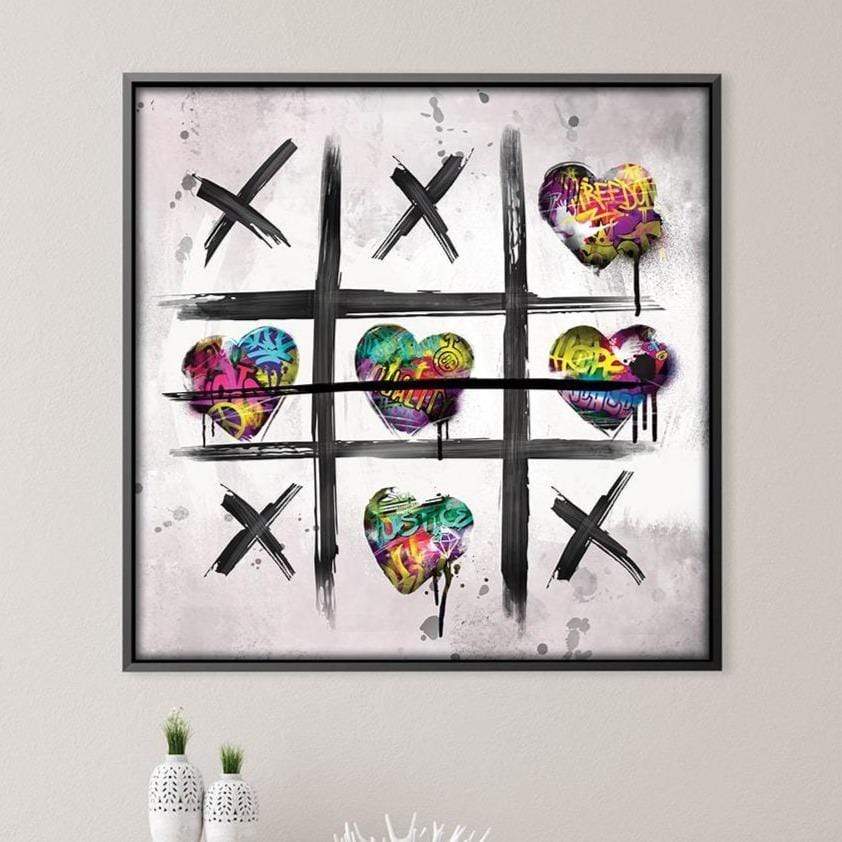This photograph features a framed piece of modern, edgy artwork displayed on a white wall. The artwork depicts an artistic interpretation of a tic-tac-toe game, presented in a square format with a black frame. The tic-tac-toe grid is created using loose, broad black paintbrush strokes, forming nine squares. Within the grid, the X's are represented by quick, black paint strokes, while the O's are depicted as vibrant, graffiti-style hearts filled with colorful words and symbols like "freedom," "hope," and peace signs. The hearts display a variety of colors, including yellow, purple, pink, blue, and green. The configuration of the game shows: X, X, heart in the top row; heart, heart, heart in the middle row (indicating a win with a bold black line drawn through it); and X, heart, X in the bottom row. The background of the artwork features gray splatters, adding to its contemporary feel. In the lower foreground of the photograph, two white vases adorned with small green and yellow plants are positioned, likely on a table just below the framed artwork.